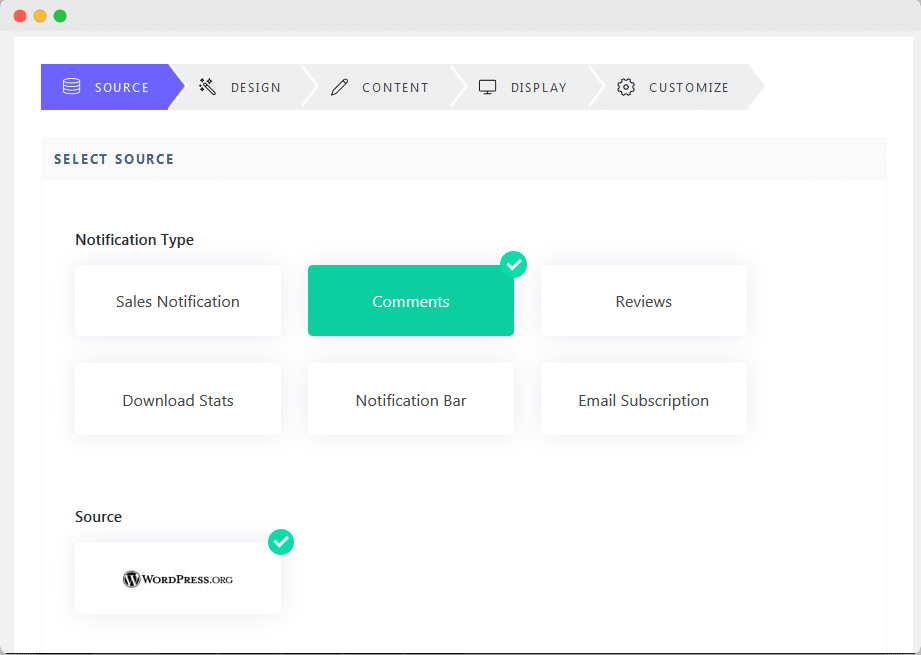The image depicts a web page interface with multiple navigation and option elements. At the top left corner, there are three small circles: one red, one orange, and one green, presumably for window control (close, minimize, maximize). Below these circles, the navigation menu includes tabs labeled Source, Design, Content, Display, and Customize.

The main section of the page is focused on selecting a source for notifications, as indicated by the "Select Source" heading. Underneath this, there is a "Notification Type" section listing various options: Sales Notification, Comments, Reviews, Download Stats, Notification Bar, and Email Subscription. Currently, the "Comments" option is highlighted in green and marked with a green check mark in the top right corner of the option button.

Towards the bottom of the page, there is another "Source" label followed by a box displaying "WordPress.org." This box also features a green check mark in a circle at the top right corner, indicating a verification or selection status. The overall layout is clean and organized, guiding the user through the process of configuring notification sources.